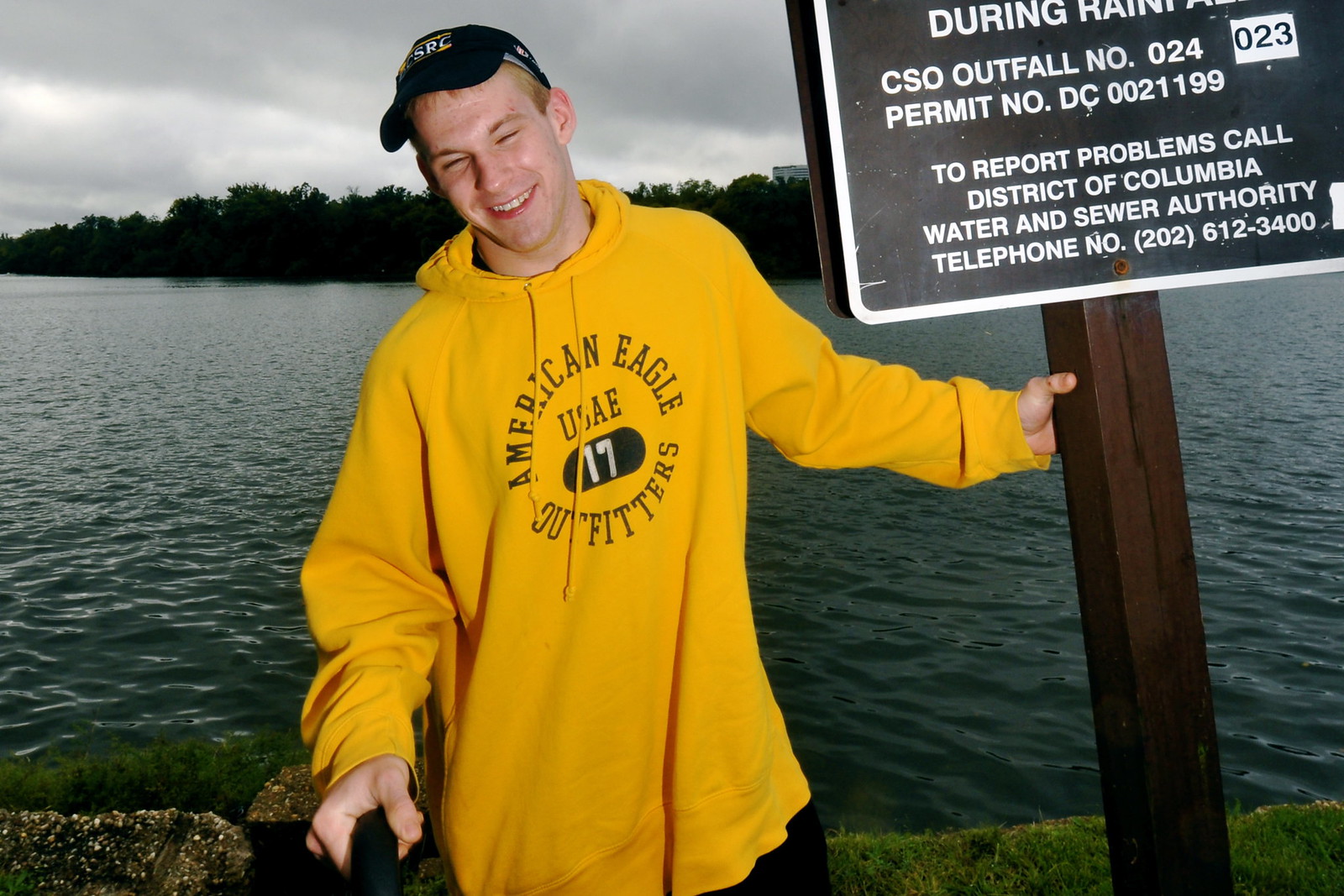The image captures a close-up of a white male in his 20s wearing a yellow "American Eagle Outfitters USA" hoodie and a black baseball cap. He stands facing the camera with a smile and his eyes mostly closed, head slightly tilted to the left. His left arm stretches out to hold a wooden pole with a partially visible black sign, displaying white text that reads, "During rain" and "CSO outfall number 024, permit number DC0021199." The sign mentions reporting problems to the District of Columbia Water and Sewer Authority and includes a contact number. The setting appears to be an overcast afternoon with a stormy, gray sky. In the background, there is a body of water, possibly a river or lake, with a wooded area of trees and bushes lining the horizon. His image is framed just below the waist, revealing a glimpse of his black pants.